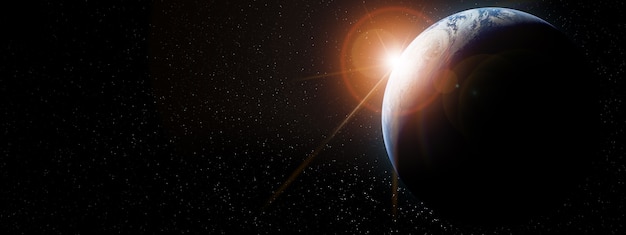In this computer-generated panoramic image of outer space, the left side showcases a vast expanse of blackness dotted with small white specks representing distant stars. Dominating the right side of the image is a large blue orb, identified as Earth, partially illuminated by the Sun positioned behind it. The Sun casts an orange glow with a lighter halo around it, sending visible rays and lens flares through the cosmic scenery. The front hemisphere of Earth is bathed in light, seamlessly transitioning to darkness on its back right half, with the star-specked void continuing behind the planet.